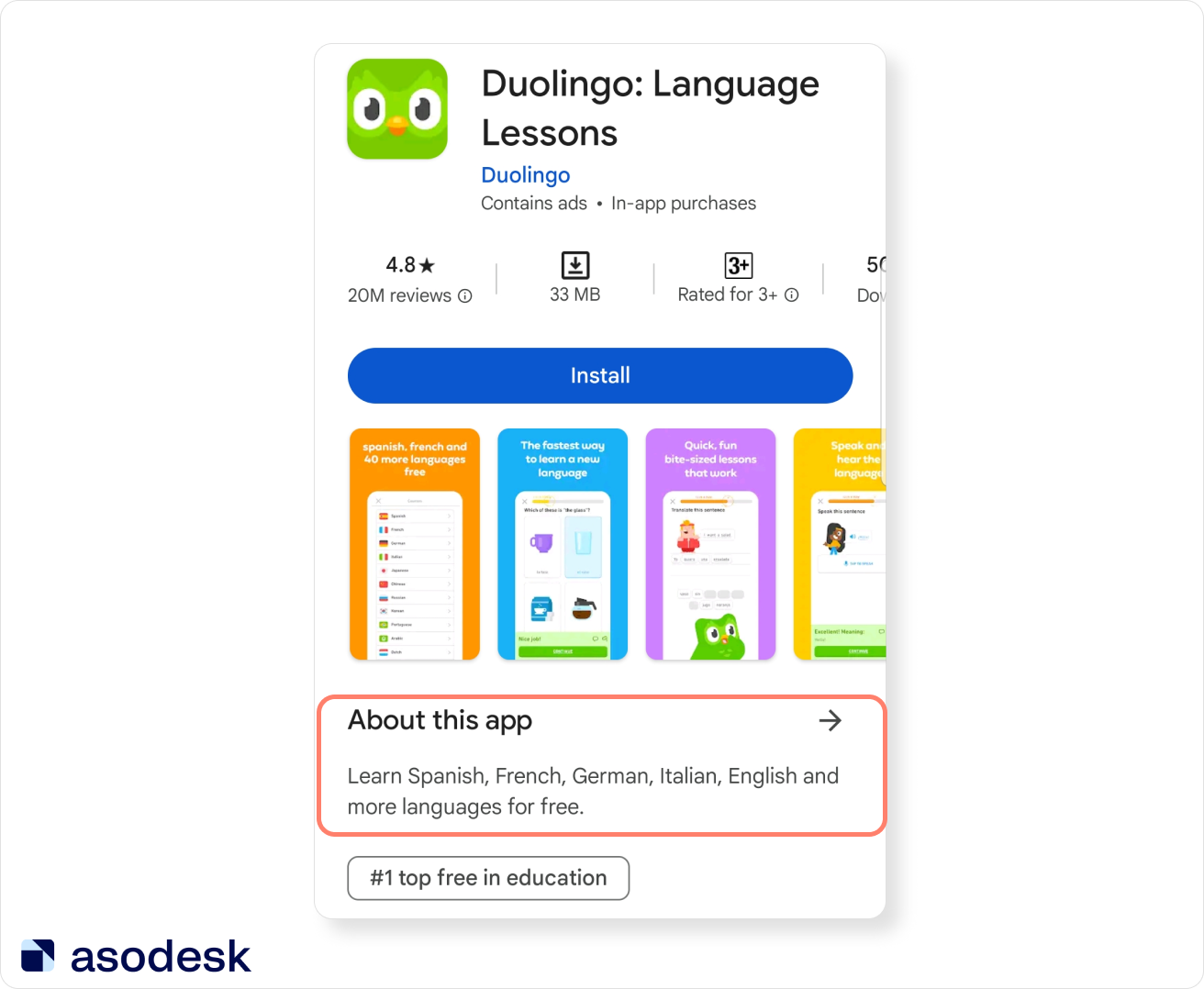This screenshot is for the app Duolingo, as displayed in an App Store listing. The background is predominantly white, providing a clean and minimalistic look. 

- **Top Left Corner**: Shows the Duolingo logo, featuring a green owl face with vivid eyes and nose.
- **Right of the Logo**: The text "Duolingo: Language Lessons" is prominently displayed.
- **Beneath the Title**: The word "Duolingo" appears again, indicating the app's developer.
- **Below the Developer Info**: A note that says "Contains ads and in-app purchases".
- **Review Section**: The app boasts a 4.8-star rating from 20 million users and highlights its compact size of 33 megabytes. Adjacent to this, an age rating indicates it is suitable for users aged 3 and up.
- **Install Button**: A blue button with "Install" written in white font is provided for downloading the app.
- **App Previews**: Four colorful screenshots below the install button give a glimpse into the app's interface and features.
- **About This App Section**: A red rectangular box spans the width of the screenshot, with "About this app" written in black font and an arrow pointing to the right.
- **App Description**: Below the red box, the text reads "Learn Spanish, French, German, Italian, English, and more languages for free".
- **Additional Box**: At the bottom, another section with a black border indicates the app's ranking: "Number 1 Top Free in Education".

The screenshot effectively communicates all key details for potential users looking to download Duolingo from the App Store.